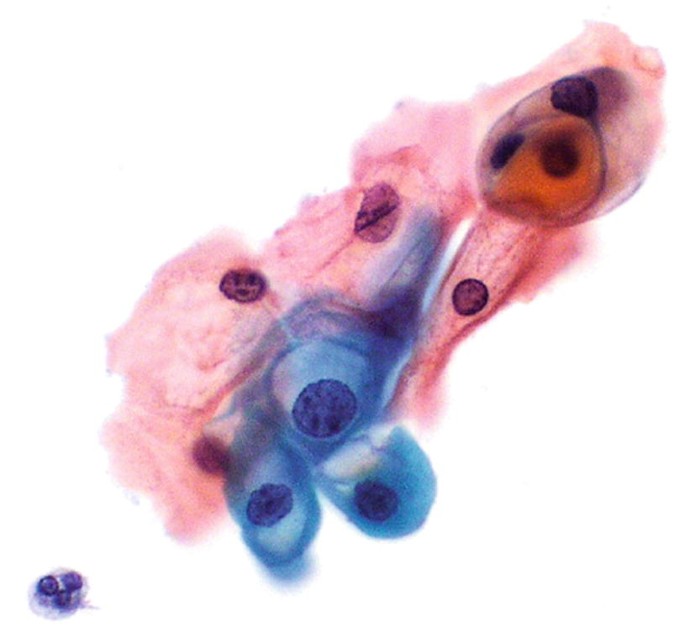The image is a vivid piece of art set against a stark white background, resembling a painted abstract inkblot. Dominated by shades of rosy pink and red, it features an organic, flowing pattern that extends from the bottom left corner towards the top right. The main body of the artwork is reminiscent of flower bulbs or even amoebas, with numerous darker reddish-orange and blue spots and bulbs sprinkled throughout. A prominent blue area intersects with the reddish hues toward the center, containing several distinct blue circles. In the bottom left corner, there is a noticeable separate area with a purple tint, suggesting a detached element from the main composition. The overall shape is oblong and abstract, evoking a sense of both biological structure and artistic flair.